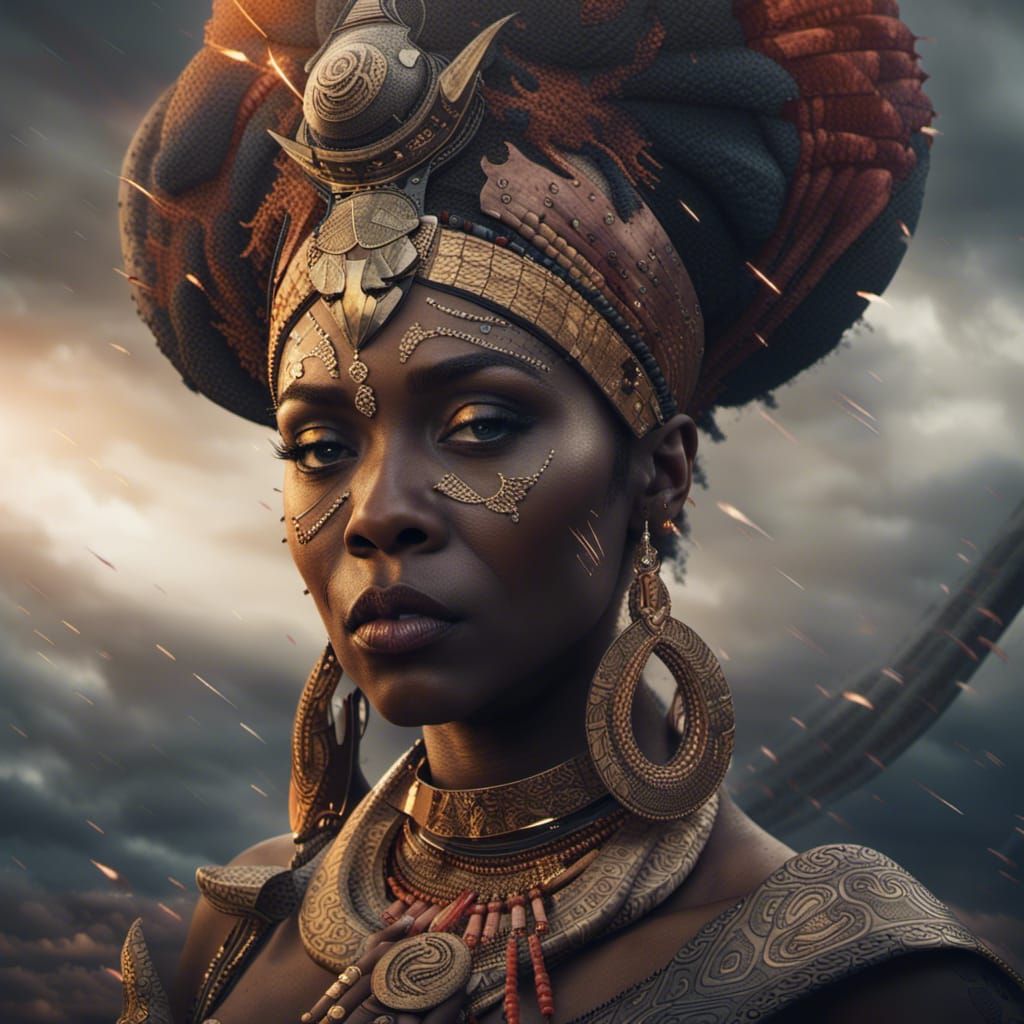This image is a beautifully detailed and realistic painting of a black woman, dressed in an Afro-fantasy style, evoking a powerful and regal presence. Her face is adorned with golden decorative items around her eyes, and she gazes at the viewers with half-closed, imperious eyes. She wears a turban, primarily blue and red, adding to her majestic appearance. Her ears are adorned with large, heavy-looking oval-shaped golden earrings that seem burdensome. Around her neck, she is showcased with layered bronze and golden jewelry, including tight-fitting necklaces and larger ornamental pieces. The background features a mix of gray and green colored clouds interspersed with yellow drops that appear to be floating, adding a dynamic and fantastical element to the scene.